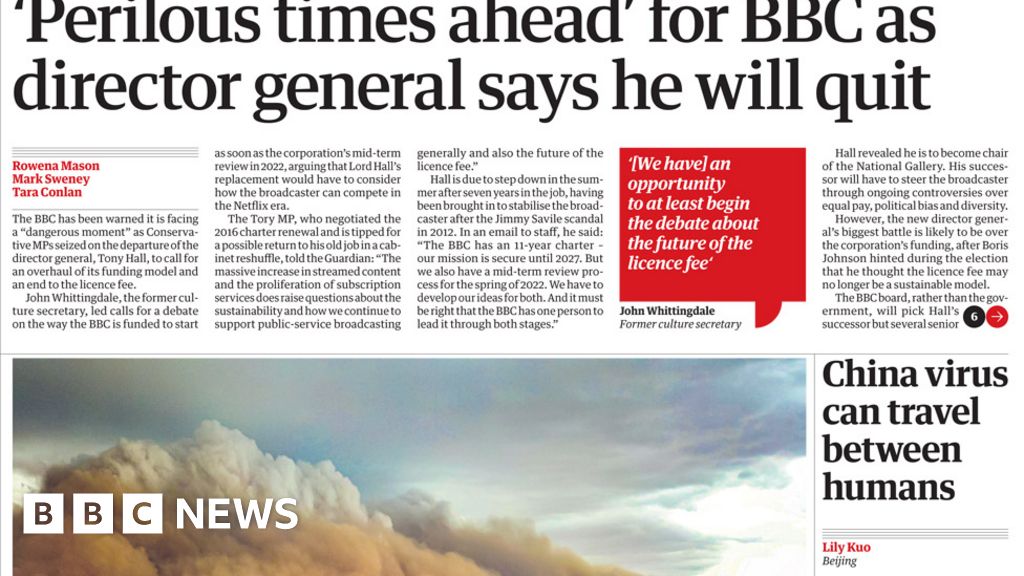An online newspaper article showcases a headline about the upcoming challenges for the BBC, alongside a variety of other news snippets. The headline reads, "Precarious Times Ahead for BBC as Director-General Announces Resignation," highlighting that Tony Hall, the current director-general, will be stepping down. Journalists Rowena Mason, Mark Sweeney, and Tara Conlan contribute to this report.

The article details the BBC’s warning about facing a critical juncture with conservative MPs exploiting the director-general’s departure to push for a reevaluation of the broadcaster's funding model, specifically by advocating for an end to the license fee.

On the right, there is a highlighted quote in red from John Whittingdale, former culture secretary, stating: "We have an opportunity, at least, to begin the debate about the future of the license fee."

Below this, there is another headline, "China Virus Can Travel Between Humans," authored by Lily Kuo in Beijing.

Accompanying these articles is a photograph of the sky filled with clouds of varying shades – gray, blue, white, and a few tinged with an orange hue, reminiscent of smoke from a fire. The BBC News logo is positioned in the bottom left corner of this image, with the letters "BBC" in white blocks, allowing the cloud-filled background to show through, all set against a black and white theme for the page’s design.